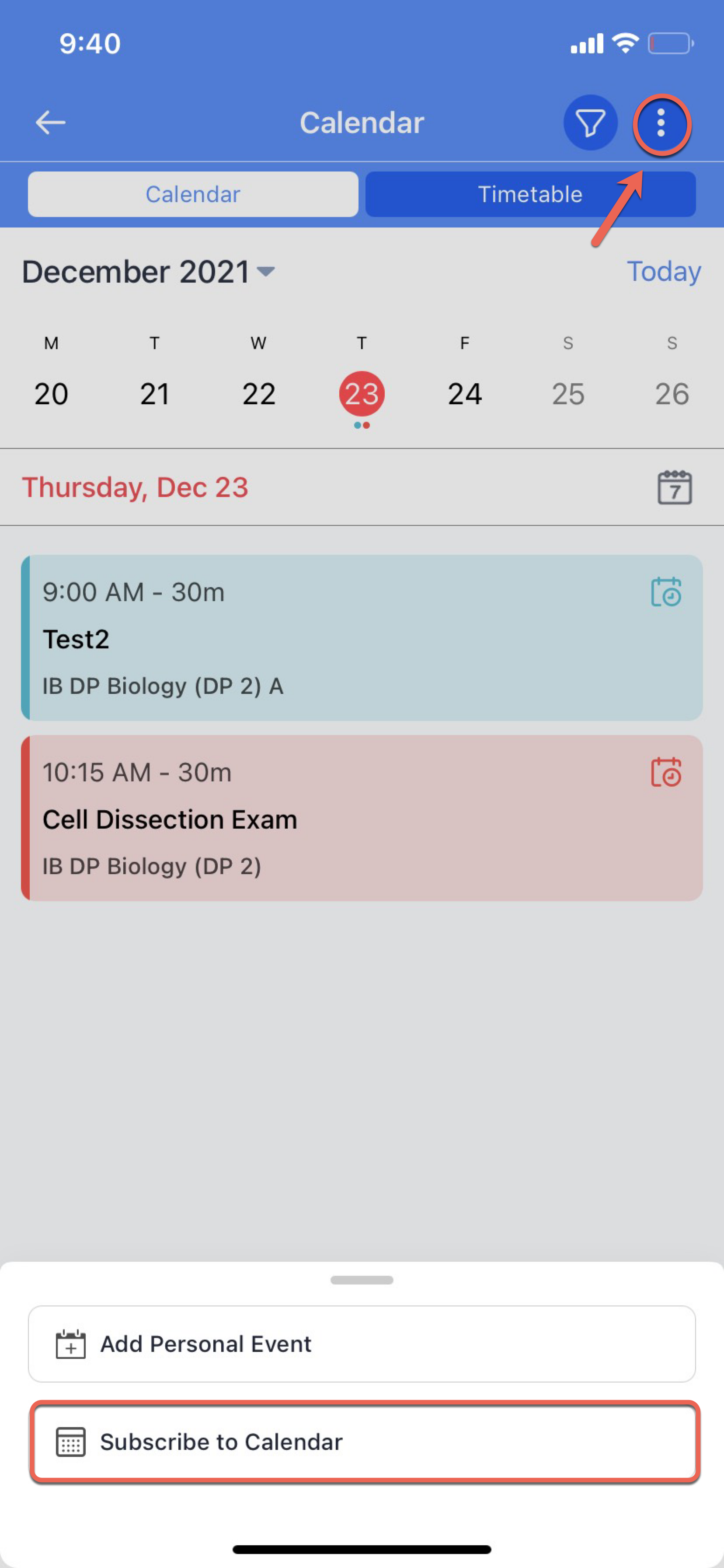This is a detailed screenshot of a calendar setting app on a smartphone. At the top right corner, a red arrow points to a vertical trio of dots, indicating a menu option. The current time displayed on the phone is 9:40 AM, with both the cell phone and Wi-Fi reception at full strength. However, the battery level is critically low.

The screen's header features the word "Calendar" prominently in the center, with a white back arrow positioned to its left. Adjacent to "Calendar" on the right, there is a filter icon followed by the red-circled three-dot menu icon previously mentioned.

Beneath the header are two selectable tabs labeled "Calendar" and "Timetable." The displayed date is Tuesday, December 23, 2021.